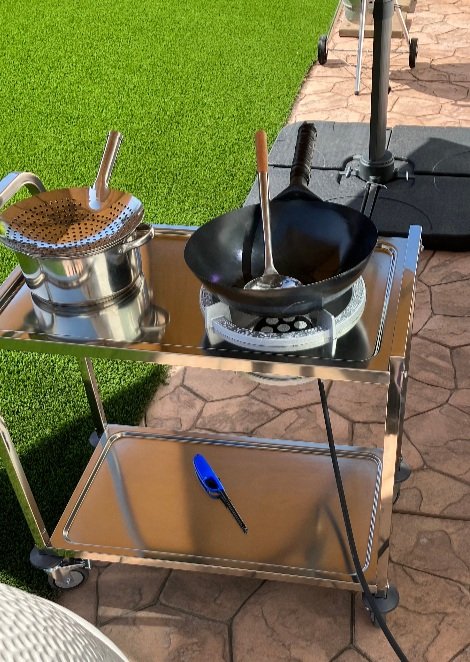This detailed photograph captures an outdoor cooking setup situated in a modern garden. Prominently placed in the center, there's a two-tiered stainless steel rolling cart. On the top tier, to the right, is a large, black wok featuring a substantial silver ladle resting inside it, positioned over what looks like coals or a heating element. To the left of the wok, there's an impressive stainless steel pot covered with a perforated steamer, likely used for steaming food.

The bottom shelf of the cart holds a long, blue stove lighter with a black tip, indicating preparedness for lighting cooking flames. The scene is set against a contrasting background; on the left side, there's green turf or grass, while the right side features tan stone pavers commonly found on patios. Additional elements include a hint of a white, textured object that might be a smoker in the bottom left corner, the legs of what seems to be a grill in the back right corner, and a black, square base with a pole that could be part of a lighting setup or possibly a pedestal for a basketball hoop. This combination of items forms a comprehensive and sophisticated cooking setup ideal for outdoor culinary activities.